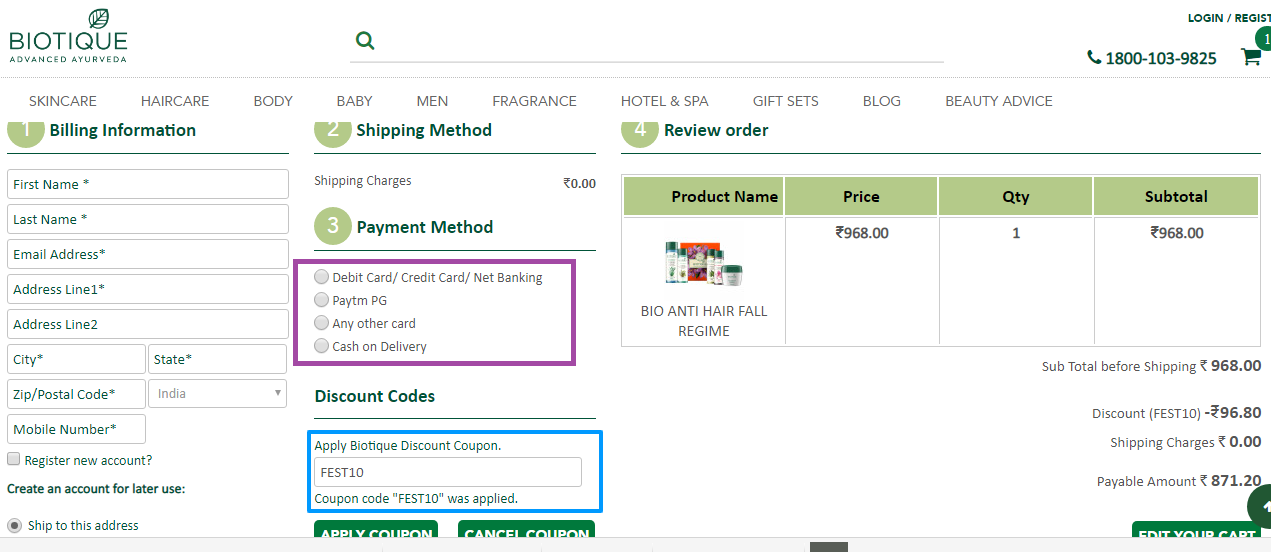This image displays a webpage for Biotic, an advanced Ayurveda brand specializing in skincare, haircare, body care, men's care, fragrances, hotel and spa products, and gift sets. Additionally, the site features a blog and offers beauty advice. 

At the top right corner of the page, there are options for Login and Register, along with a customer service phone number: 1800 103 9825. The webpage guides users through a checkout process which is divided into four main sections: 1) Billing Information, 2) Shipping Method, 3) Payment Method, and 4) Review Order.

Under the "Billing Information" section, users are prompted to enter their first name, last name, email address, address line 1, address line 2, city, zip or postal code, state, and mobile number. There are also options to register a new account, create an account for future use, and choose to ship to the billing address.

The "Payment Method" section provides multiple options for completing the purchase, including debit card, Paytm, Paygee, other cards, and cash on delivery.